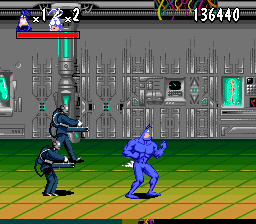This image is a screenshot from a 2D side-scrolling video game. At the center of the graphic is the main character, outfitted in a distinctive blue suit. On the left-hand side of the screen, two enemies in dark, possibly black suits are approaching, both pointing their guns towards the protagonist, creating a sense of imminent danger. In the top left corner of the image, there is a red health bar indicating the character's vitality, currently showing 'one life, two lives'. Just below the health bar is the player's score, which reads '136440'.